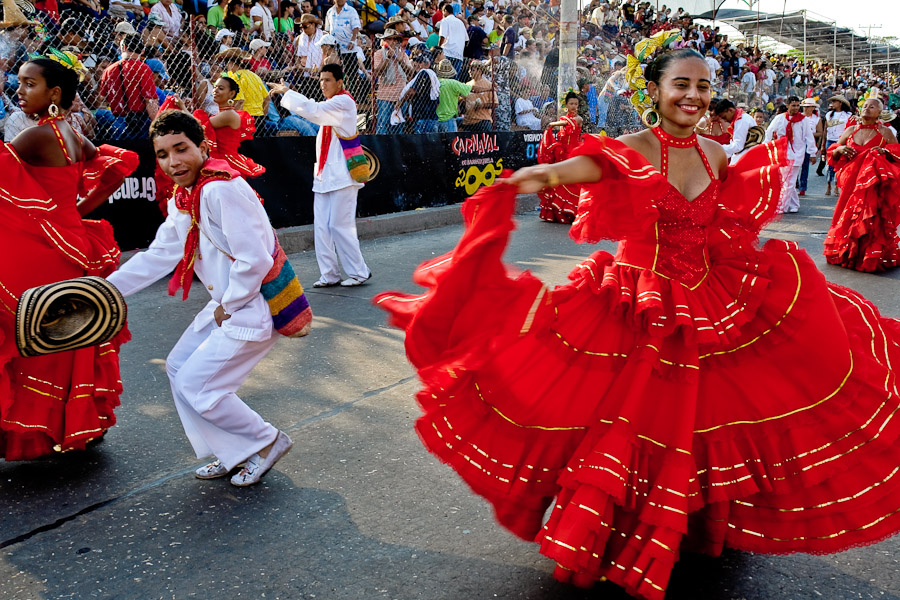This full-color photograph captures an outdoor daytime scene at a lively carnival or festival, specifically Carnival 2005, as indicated by the sign on the bottom of the fence. The scene is set on a gray pavement in front of a crowd seated in tiered stands that ascend in height, all enclosed by a chain-link fence. 

Central to the image is a dynamic group of dancers adorned in striking ethnic attire. The male dancers are uniformly dressed in pristine white ensembles, including long-sleeved shirts, pants, and shoes, each accentuated by a red scarf around their necks, and they carry colorful hats instead of wearing them. A male dancer can be seen towards the left side of the image holding a vividly patterned bag.

The female dancers are attired in eye-catching, off-the-shoulder red dresses that flow elegantly around their ankles, embellished with white and gold lines, ruffles, and bell-shaped bottoms. Their hair is neatly pulled back into decorated buns featuring yellow and green adornments, and many wear large hoop earrings. A prominent female dancer, positioned on the right side of the image, nearly spans the photo from top to bottom.

All the dancers appear to be engaged in animated dance movements, contributing to the festive and energetic atmosphere of the occasion, with more female dancers visible in the background.